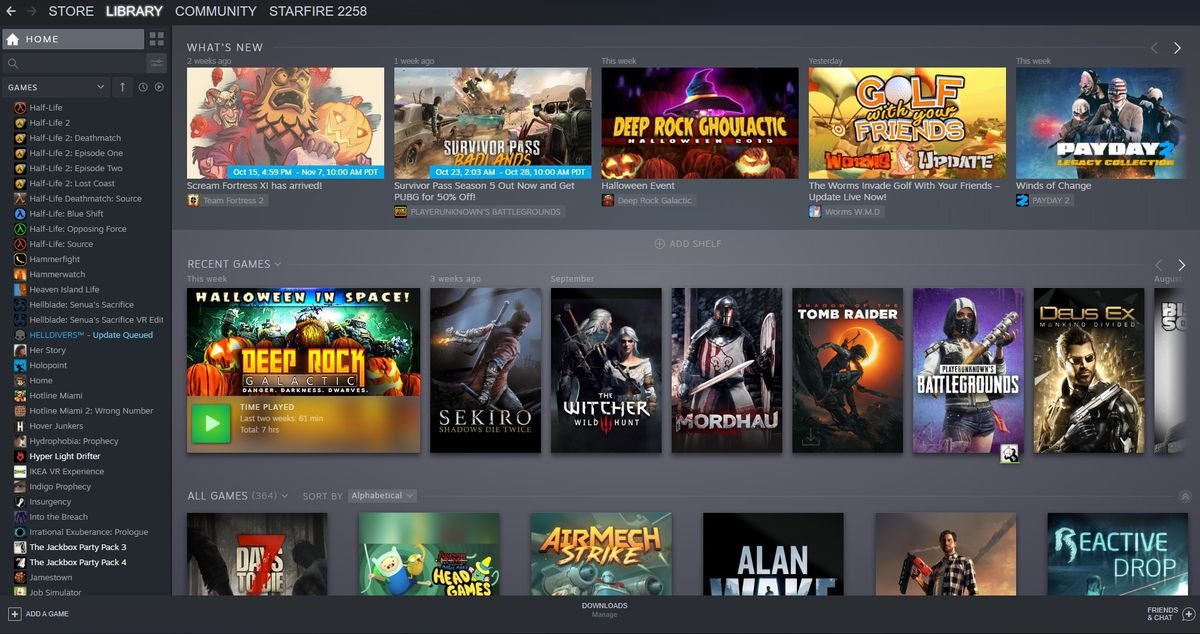This detailed caption provides a clear, concise, and engaging description of the image:

---

The image captures a screenshot of the front page of a gaming application called Stream. At the top left corner, there is a navigation bar that includes a back button, a home button, and four clickable links labeled Store, Library, Community, and Starfire 2258. Dominating the central section of the page are several cover images of various video games, including prominent titles such as Tomb Raider, The Witcher, and Air Merch Strike. To the left side of the page, a long, scrolling list of video game titles is visible, extending from the top to the bottom of the screen. The overall background color of the application is a sleek shade of gray. This screenshot effectively showcases the interface and design elements of the Stream gaming platform.